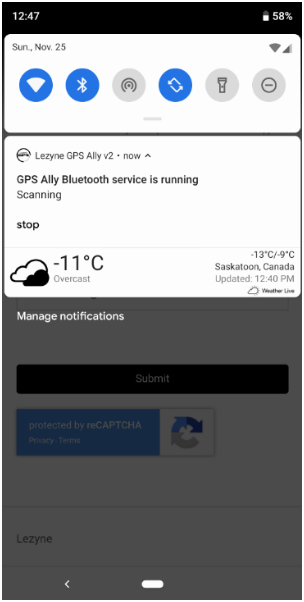The screenshot captures a notification panel on a mobile phone displaying a predominantly white user interface. At the top, there are six circular icons aligned horizontally. The icons represent Wi-Fi, Bluetooth, signal strength, screen rotation, a torch, and a minus symbol respectively. The Wi-Fi, Bluetooth, and screen rotation icons are highlighted in blue circles with white symbols, indicating they are active. The signal strength, torch, and minus symbol icons are in gray circles with darker gray symbols, indicating they are inactive.

Directly below these icons, a notification reads "GPS Allied Bluetooth service is running" followed by the word "scanning." Just below this message, there's a "stop" option likely intended to halt the scanning process. Further down, a white and black cloud icon is present, next to which it displays the temperature as "minus 11°C." At the bottom of the notification panel, there's an option labeled "Manage notifications" written in white text, allowing users to configure their notification settings.